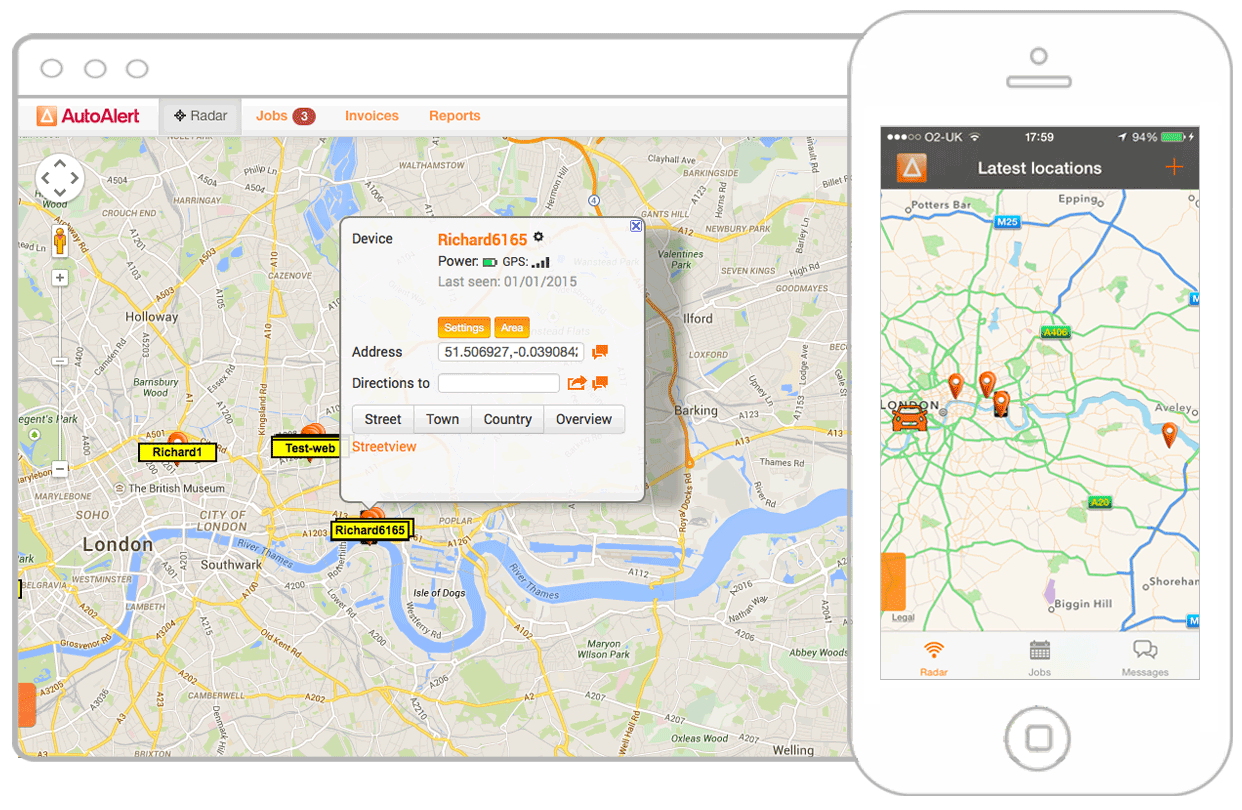Here is a detailed and cleaned-up caption for the described image:

---

This image depicts a detailed mock-up commonly found in app stores like the Apple Store or Google Play Store, showcasing an app interface as it would appear on a smartphone. On the right side, the mock-up features a white-bordered silhouette of a smartphone with a predominantly white background, highlighting the app's visual elements. The central display shows a map excerpt powered by AutoAlert.

At the top of the smartphone mock-up, typical iPhone status indicators are shown, including a three out of five signal strength bar marked "G2 UK," a Wi-Fi symbol, the time displayed as "17:59," and a battery icon at 94% indicated in green. An orange square with a triangle icon is prominently featured, labeled "Latest Locations" in white, positioned centrally. Adjacent to this is a small orange plus sign. The map is rendered in tan, with green lines representing highways and blue lines denoting waterways. The map is dotted with multiple pins. At the bottom of the mock-up, the home button is illustrated as a circle enclosing a square.

On the left side of the image, the mock-up is shown within a web browser, or possibly as a zoomed-in close-up. The header reads "AutoAlert" accompanied by an orange square and a white triangle. The "Radar" tab is selected, displaying the map with various orange pins and yellow rectangles bordered in black, each labeled with text like "Richard-1," "TestWeb," and "Richard-165," likely indicating hand radios or radio stations. Additionally, the image showcases a "Jobs" tab highlighted with a red circle containing the number three, and features sections labeled "Invoices" and "Reports."